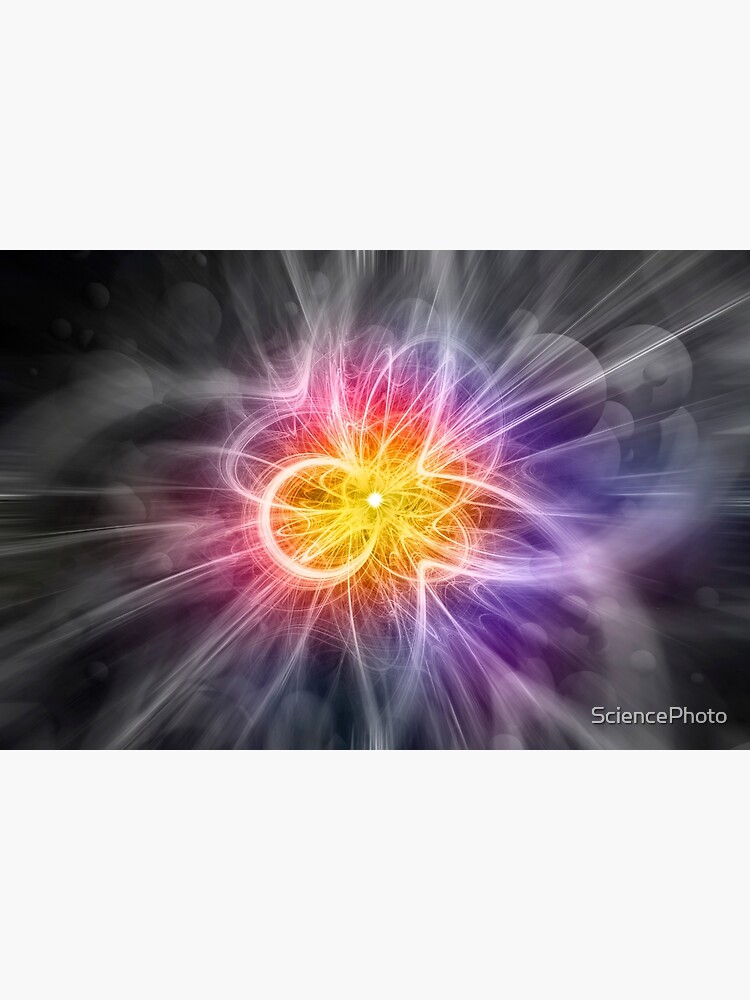This detailed 3D-generated image features an abstract composition that appears to illustrate a scene on an atomic or astronomical level, with a label in white sans serif text at the lower right corner reading "science photo." Central to the image is a bright, shiny, white object, from which emanate numerous vibrant, swirling lines resembling neon streaks. These lines, numbering in the hundreds, create oval and circular patterns that suggest rapid motion or orbiting. They transition through a spectrum of colors from yellow at the origin, to red, pink, and finally purples and oranges, creating a mesmerizing rainbow effect. The backdrop is primarily dark gray to black, accentuating the luminous swirls and lending depth to the scene. Scattered throughout the background are black and white spherical objects of various sizes, which float and add to the visual complexity. This intricate composition blends scientific imagery with an abstract aesthetic, capturing both an energetic and dynamic essence.